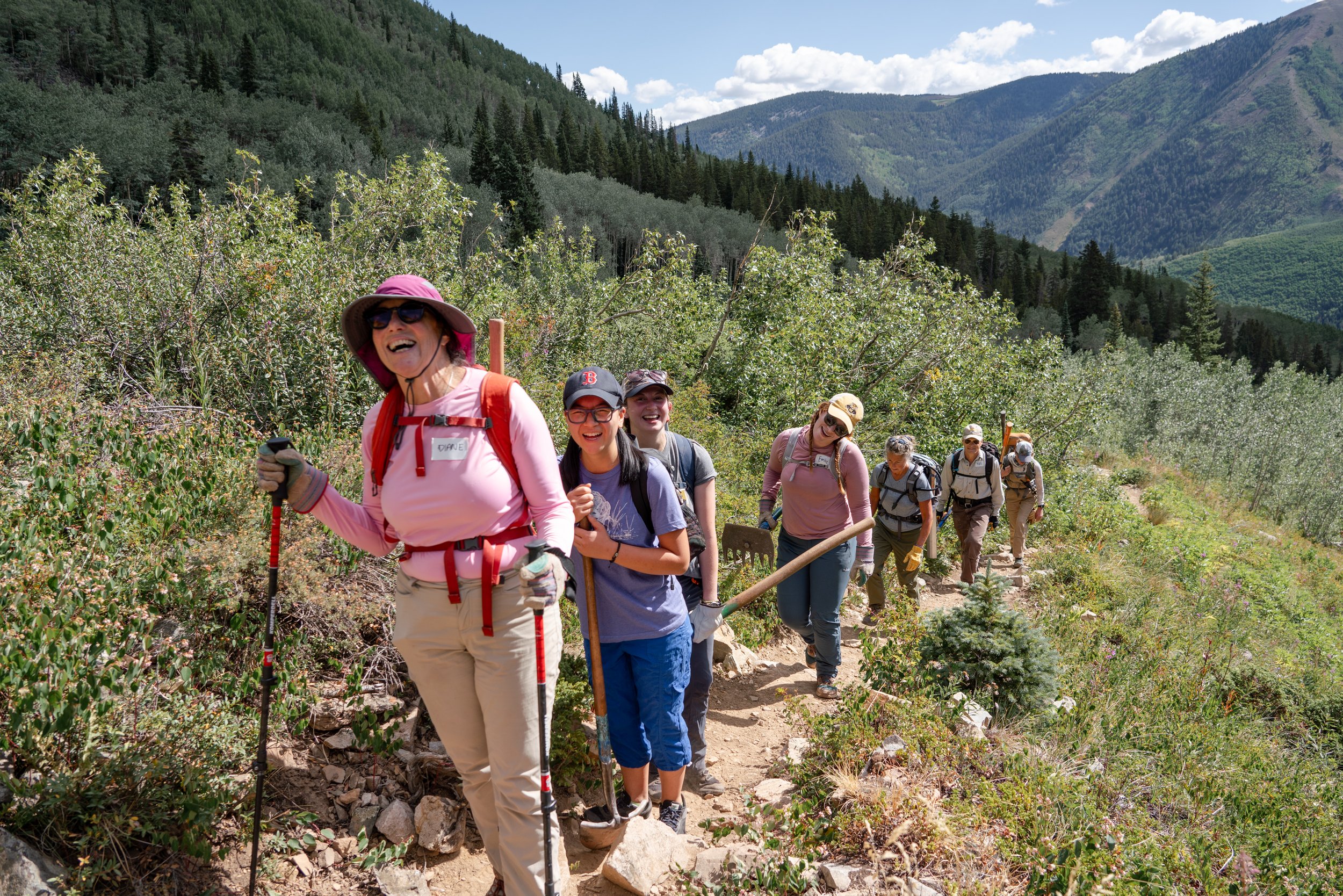This detailed photograph captures a vibrant scene of a group of eight hikers traversing a well-trodden dirt trail on a mountainside, surrounded by lush green brush and towering trees. The trail, which has been cleared by frequent use, features a smattering of large rocks on either side, adding a rugged texture to the terrain. The sky above is a bright, light blue, adorned with large, puffy white clouds. 

Leading the group is an older woman, Diane, easily identifiable by her all-pink attire, including a pink long-sleeved top, hat with a pink band, brown gloves, and brown pants. She confidently uses hiking poles in both hands and wears a wide smile, a name tag, and a bag tied around her waist with a red strap. Directly behind her is a young Asian individual donning a blue ball cap with a red "V," clear lens glasses with black frames, a short-sleeved light blue t-shirt, and rolled-up dark blue pants. They too are smiling at the camera, embodying the joyous spirit of the hike.

Further back in the line, another man, holding a handle of an indistinguishable tool, and another hiker wearing a pink long-sleeved top and blue pants wielding a large rake, add to the diverse equipment the group is carrying. Each hiker is equipped with a backpack, and some utilize hiking poles for stability. This diverse group, including at least one young man holding a shovel, appears well-prepared for their journey through the open wilderness.

In the mid-ground, beyond the hikers, rolling hills and distant mountains create a picturesque backdrop, covered in vibrant greenery that contrasts beautifully with the trail's earthy tones. The scene is a harmonious blend of human adventure and natural beauty, encapsulating the essence of a communal outdoor experience.